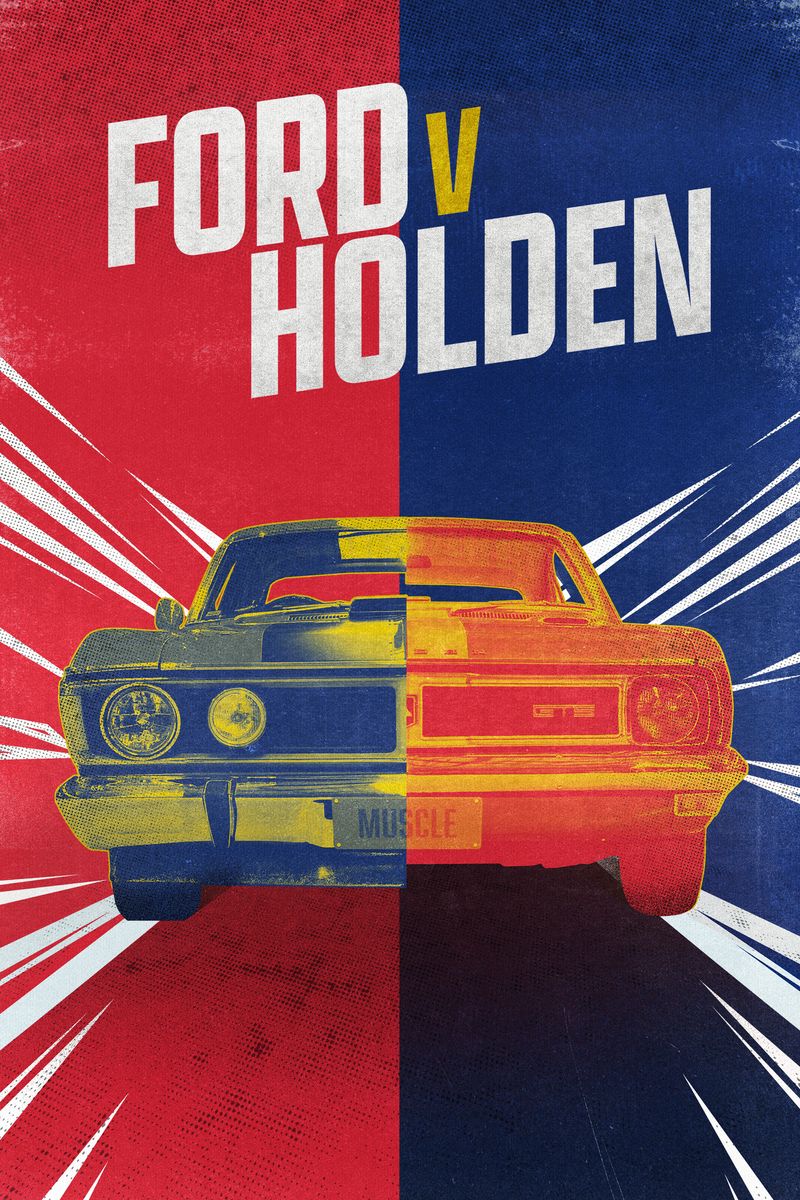This poster is split vertically into two distinct halves: the left with a red background and the right with a mix of light and dark blue. At the top, bold white text reads "Ford V Holden" with a yellow "V." The focal point is a muscle car from the 1960s or 1970s, positioned in the center and pointing straight at the viewer. The car is rendered differently on each side: on the left, against the red background, it appears in bluish hues with yellow highlights; on the right, against the blue background, it is shaded red with orangish-yellow highlights. White streaks radiate from the car, enhancing its prominence. The front license plate reads "MUSCLE," and the grill features the letters "GTS." The car's color variations and split design may symbolize the rivalry between Ford and Holden, although the exact reference is unclear.